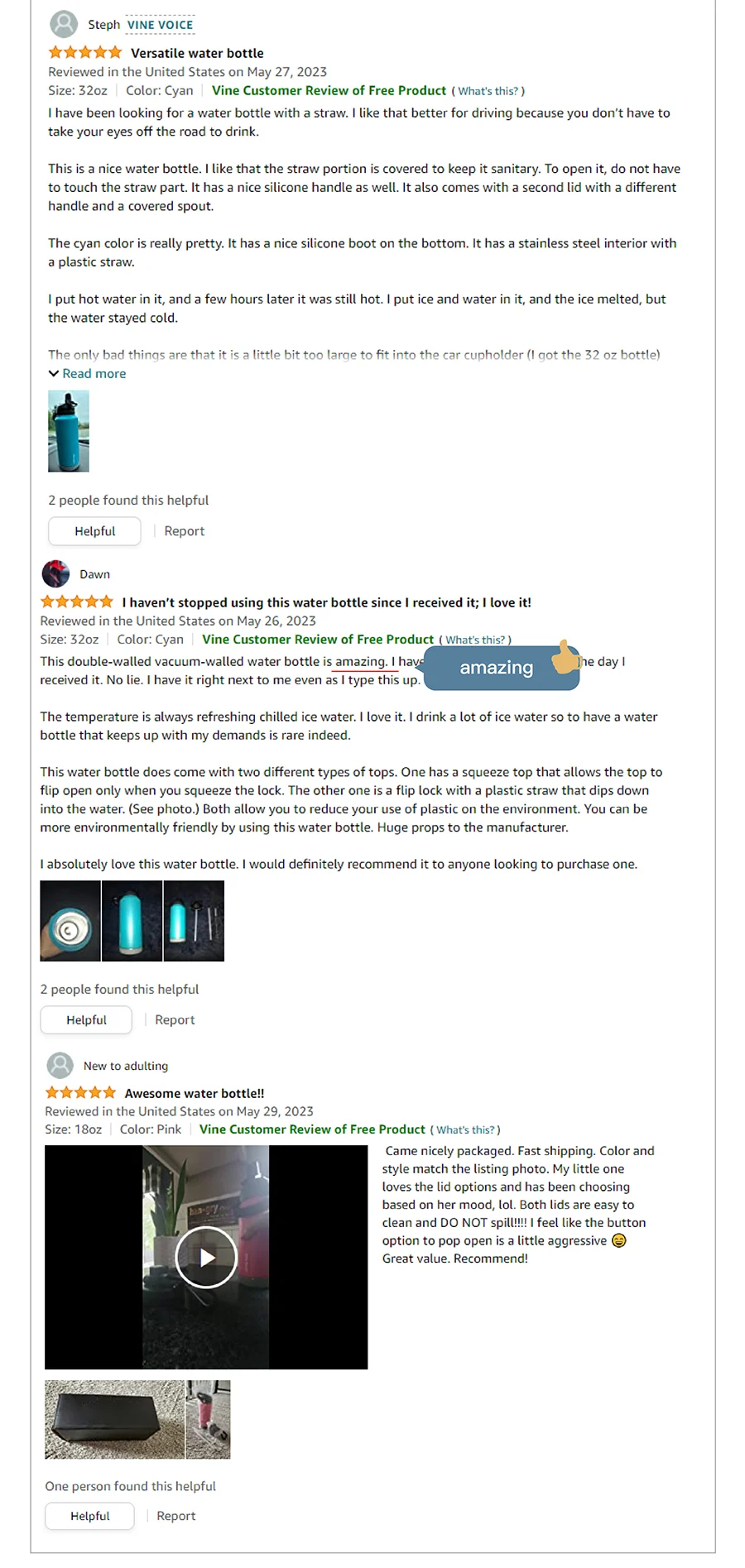The image showcases an Amazon review page with the characteristic layout, including familiar elements such as dark green text stating "View customer review of free product," orange star ratings depicting a five-star scale, and gray user icons with white detailing. In the upper left corner, a review by a user named Steph is presented. The name "Steph" appears in a small, bold, black, sans-serif font. Adjacent to this, "Vine Voice" is highlighted in dark blue, bold, capital letters with two matching blue lines bordering the top and bottom.

Although the review text is too small to read, it is evident that Steph included an image in the review, as a thumbnail at the bottom depicts an outdoor scene. Below this, there is text stating "2 people found this helpful" in black. The "Helpful" button is designed with a white background, dark gray border, and black text within an oval-rectangular shape next to a vertical divider labeled "Report."

Another review by a user named Dawn is partially visible. Dawn's profile picture is small and unclear. The review boasts a perfect five-star rating, indicated by all five stars marked in orange. Superimposed on Dawn's review is an oval with a rectangular touch, featuring the word "Amazing" in white lettering against a Navy blue background, accompanied by a thumbs-up symbol.